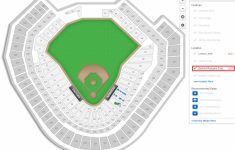This image is a graphic representation of a baseball field, with the image being wider than it is tall. The graphic is not very large and features a noticeable white background, which causes it to blend into its surroundings. Despite being fuzzy, the image clearly depicts a green baseball field. The field includes distinct brown areas marking the infield and the pitcher’s mound. Surrounding the field are outlined sections representing the stands, which are segmented into boxes. These boxes are numbered similarly to track housing and encircle the baseball diamond.

The seating sections are marked in three color-coded rings: the innermost ring is a light gray or nearly white, the middle ring is a darker gray, and the outermost ring is the darkest gray, all encased within a boundary. On the right-hand side of the graphic, there’s a box containing various lines, though the text is too small to read. A red rectangle highlights one of these lines, indicating a selection. This suggests that the graphic is likely part of a webpage for purchasing tickets to a baseball game, allowing users to select their seats within the stadium.